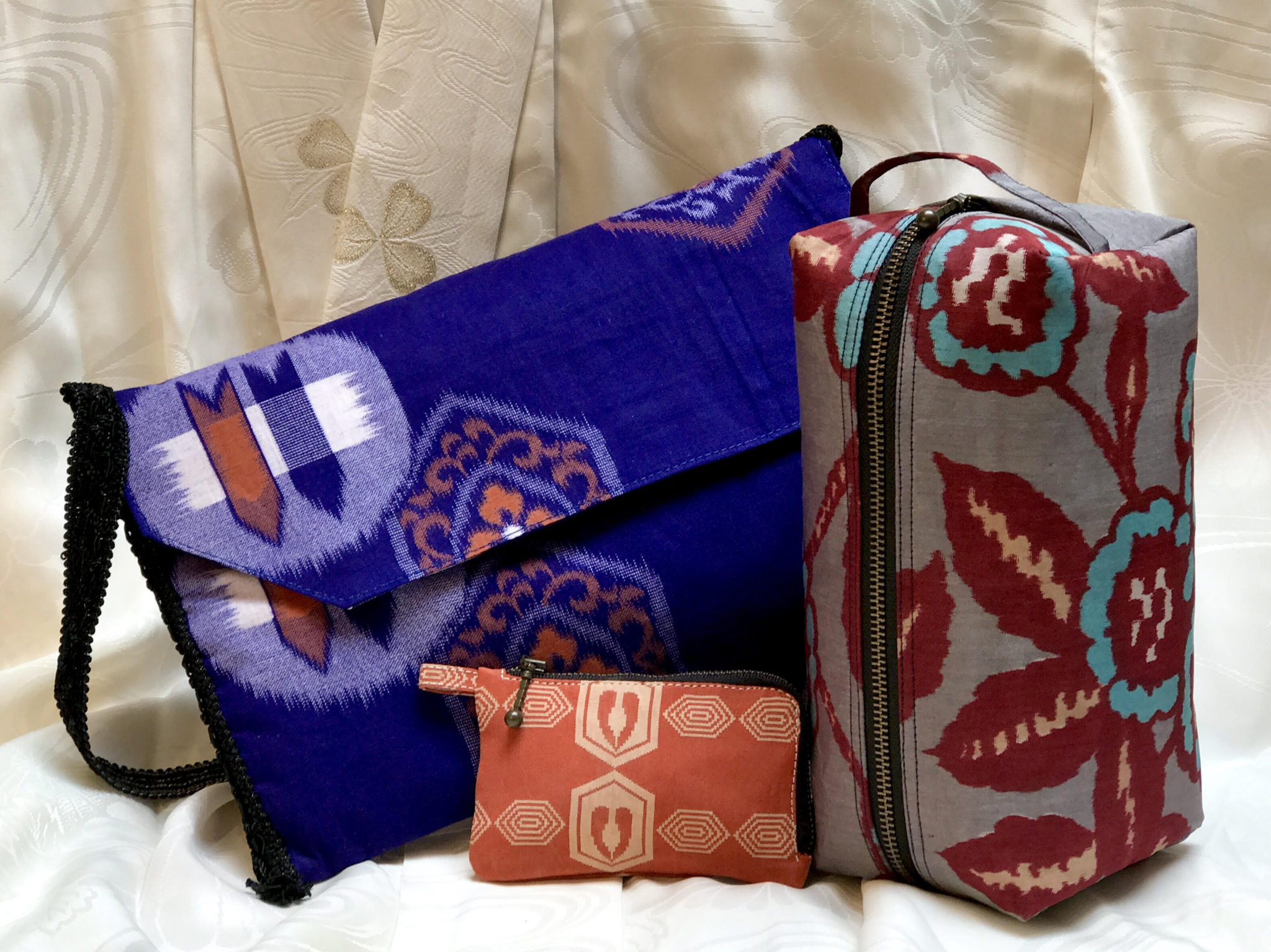The image showcases a collection of three handbags arranged on a lightly patterned, white duvet. The background features sandy-colored fabrics adorned with light flower patterns. 

The first bag is a large satchel in dark blue, accented with a blue, white, and orange design. It features a black handle and a Velcro flap closure. 

In front of it is a smaller rectangular coin pouch in a peach or light orange hue, adorned with a pattern resembling two shoe prints forming a heart-like shape and a horizontal eyeball-like design. 

To the right, there's a larger light gray bag with a zip closure, decorated with red and blue flowers and a touch of cream color.

Despite the handmade appearance of the set, the patterns and colors are distinct and do not coordinate with each other.